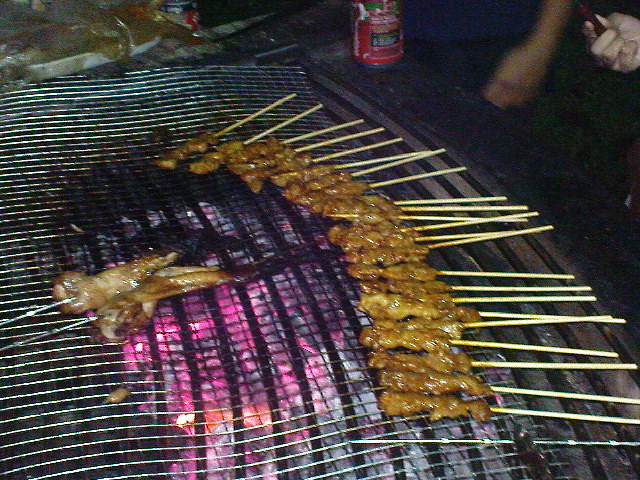This color photograph, likely taken at night, captures a large grill glowing with red hot and gray coals beneath wire grating. On the grill, approximately two dozen thin brown skewers are neatly lined up, their pieces of meat glazed to a shiny golden brown, suggesting they are chicken and nearly done. The scene is set outdoors and includes details like a reddish drink container, possibly a can of beer or soda, situated on a table surface in the upper right-hand corner. Partially visible in the same corner are two hands, one appearing blurred due to movement, hinting at people engaging near the grill. The dim, atmospheric lighting emphasizes the inviting warmth of the cooking fire.